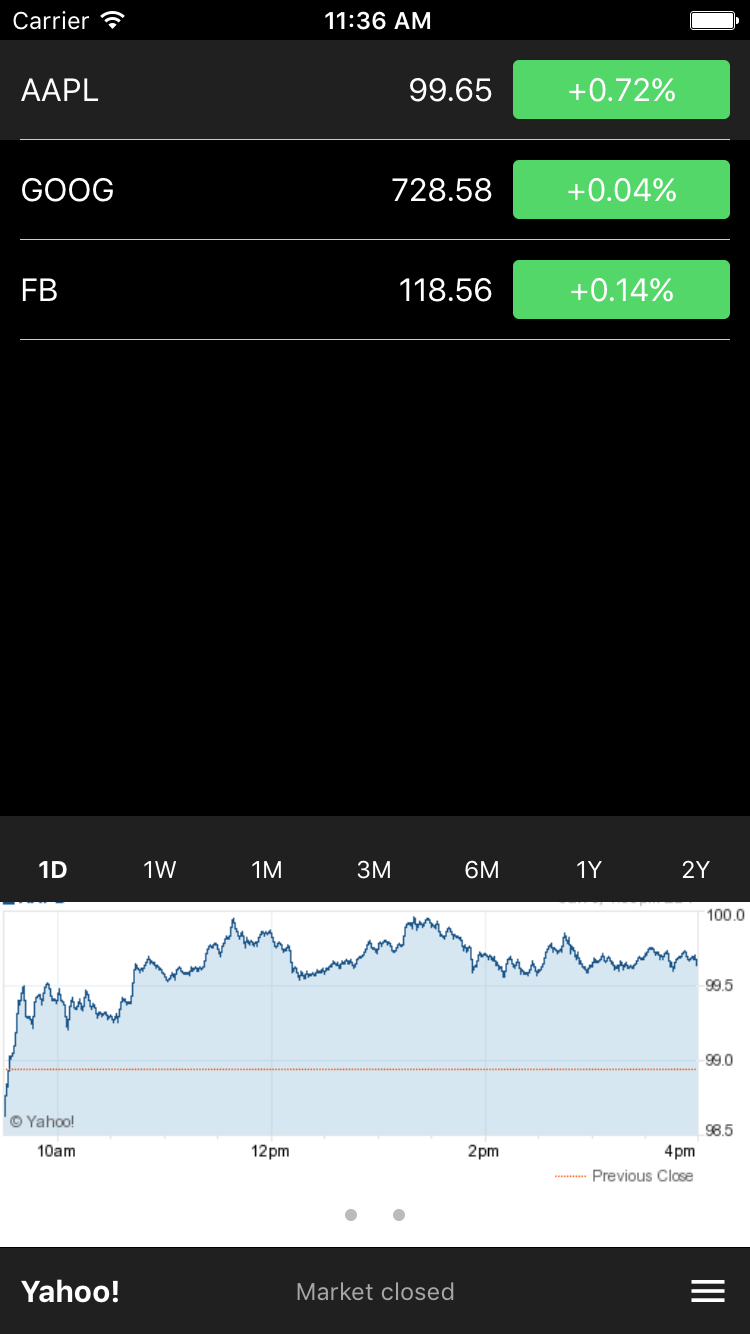This image appears to be a screenshot taken from a smartphone, displaying stock market information in an app. 

At the very top, the screen has a black background with a white status bar. This bar contains the word "carrier" on the left, the time "11:36 AM" in the middle, and a fully charged battery icon on the far right.

Below the status bar, the screen is divided into three sections by white lines. The first section, set against a light gray banner, displays "AAPL" in capital letters and the stock price "99.65". To the right, there is a green square indicating a percentage gain of "+0.72%".

The second section has a black background featuring "GOOG" in capital letters along with the stock price "728.58". Adjacent to this, a green button shows a minor gain of "+0.04%".

The third section, also with a black background, lists "FB" in capital letters followed by the stock price "108.56". A green button next to it shows a gain of "+0.14%".

Below these sections is a large black area, which contains clickable time intervals for stock performance: "1D, 1W, 1M, 3M, 6M, 1Y, 2Y". 

Below this, a graph on a white background is displayed, with a blue line indicating stock performance over time. The x-axis is labeled with time markers "10 AM, 6 PM, 12 PM, 2 PM, 4 PM". A red vertical line runs down the middle of the graph.

At the very bottom, there is a black banner displaying the word "Yahoo" in white text. In the middle, it reads "Market Closed," indicating the current state of the stock market.